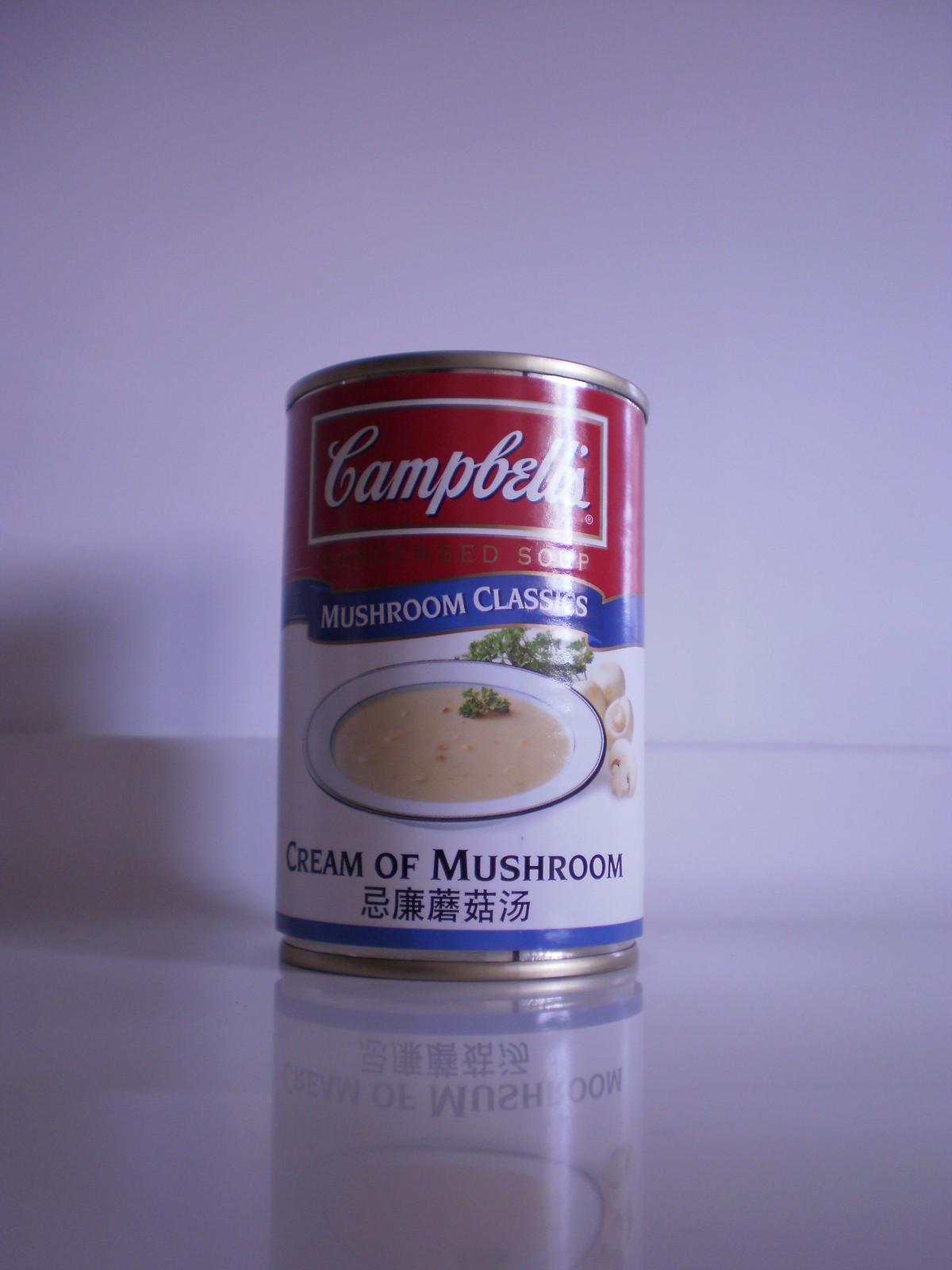This image showcases Campbell's Mushroom Classics Cream of Mushroom Soup. The can is prominently displayed in the center, featuring its distinctive red label with white text. At the center of the can, a blue label highlights "Mushroom Classics" in white lettering, while the bottom label specifies "Cream of Mushroom." Additional text, possibly in Chinese or Japanese, is present near the bottom. The can also features a blue ring at the base. Positioned in a white bowl, the creamy soup is shown on a reflective surface that mirrors the soup's appearance. The background of the image is a pristine white wall. Moreover, there is a white rectangular text box on the label containing the Campbell's logo and the website www.campbellsoup.com.